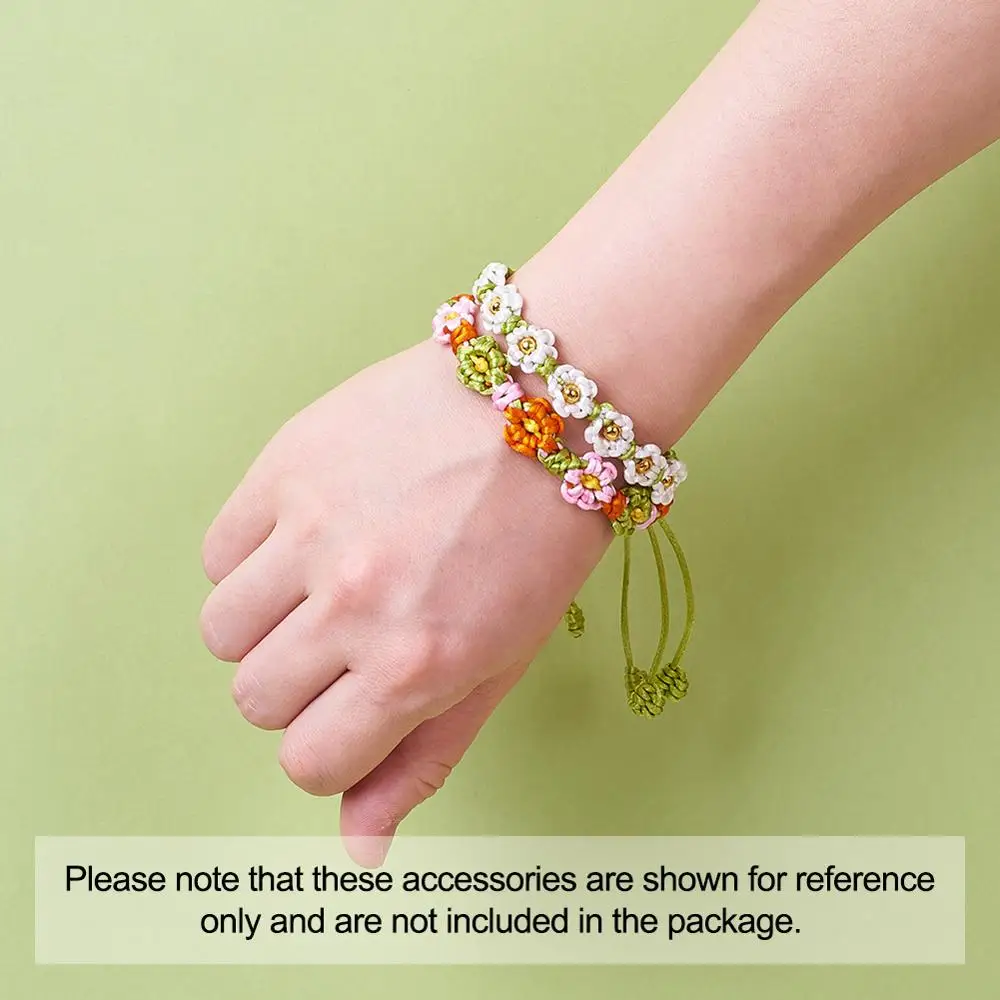A detailed image shows a peach-colored, white-skinned right arm extending from the upper right corner with the hand positioned palm-down and fingers bent at the knuckles so that the fingertips touch the palm, with the thumb pressed tightly against the fingers. The background is a blurry, pale sage green. Adorning the wrist are two delicate, green string bracelets adorned with pastel flowers in white, pink, and orange. The floral patterns have white petals with some featuring golden centers. At the bottom of the image, a white rectangular box with black lettering states, "Please note that these accessories are shown for reference only and are not included in the package."